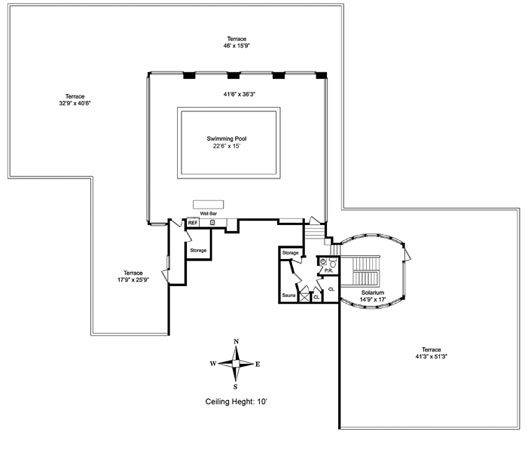This blueprint meticulously illustrates the design of a sprawling residential property, primarily rendered in light gray with accentuating black lines. The highlight of the layout is an extensive terrace that wraps around the building in an L shape, extending further out in the back to encircle the house. The rear of the property features a generously sized swimming pool, measuring 22'6" by 15', enclosed within a designated fenced area. Adjacent to this space, there is a small storage room accompanied by what appears to be bathroom facilities.

Entryways lead from the terrace into a solarium, which is also surrounded by the expansive terrace, enhancing the indoor-outdoor living experience. The blueprint includes a directional star indicating north, south, east, and west, ensuring accurate orientation. Notably, the ceiling height throughout the house is marked at 10'. Furthermore, near the solarium, there is an additional area designated for storage and a sauna, emphasizing the luxurious amenities. Doors from this section provide direct access to the pool, seamlessly blending relaxation and functionality.